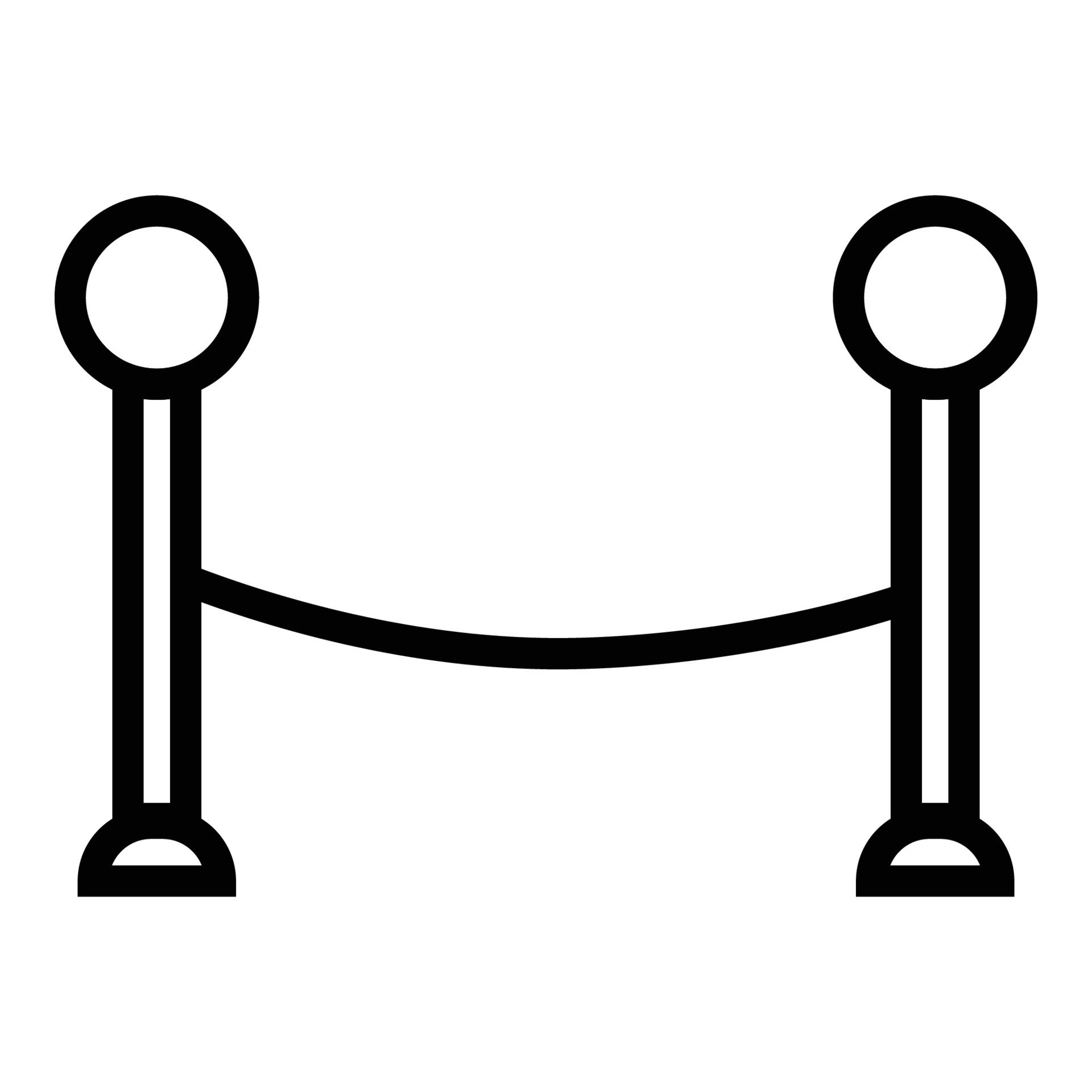The image is a minimalistic black and white illustration capturing a simple scene reminiscent of event barriers typically seen at high-class or organized settings. The background is entirely white, providing a stark contrast to the objects portrayed. In the forefront are two posts, each consisting of a semi-circular base outlined in thick black lines, supporting a thin rod extending upwards, capped by a small circle at the top. The two posts are spaced apart and connected by a single black line, which slightly curves downwards, emulating the appearance of a rope. This creates the visual impression of a barrier typically used to guide crowds or restrict access, similar to those seen at movie theaters or upscale events. The illustration’s simplicity effectively emphasizes the essential elements of the scene without any additional distractions.